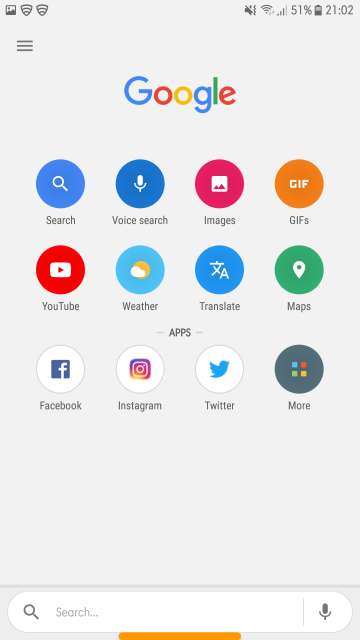The image displays a cell phone screen with a light gray background. In the top left corner, three small icons are visible: a square and two shields. To the right, an assortment of symbols includes the vibration symbol and the network strength indicator showing three out of five bars. Below this, the battery percentage reads 51%, accompanied by an upright battery icon, and the time is indicated as 21:02.

Below the status bar, in the left section of the next line, there are three horizontal gray lines. Centrally located underneath this, the word "Google" is displayed in its characteristic colors: a capital 'G' in blue, a lowercase 'o' in red, another lowercase 'o' in yellow, a lowercase 'g' in blue, a lowercase 'l' in green, and a lowercase 'e' in red.

Further down, the screen showcases 12 application icons arranged in three rows, each containing four round icons. The icons in the first row include "Search," "Voice Search," "Images," and "Gifts," listed from left to right. The second row features "YouTube," "Weather," "Translate," and "Maps," also from left to right. Between this row and the third row, the word "Apps" is displayed in small letters at the center of the screen.

The third row features icons for "Facebook," "Instagram," "Twitter," and "More," listed from left to right. At the very bottom of the screen, there is a large white oval-shaped search field. On the left side of this search field is a magnifying glass icon, while the word "Search" is typed out in light gray letters. On the far right of the search field, there is a microphone icon.